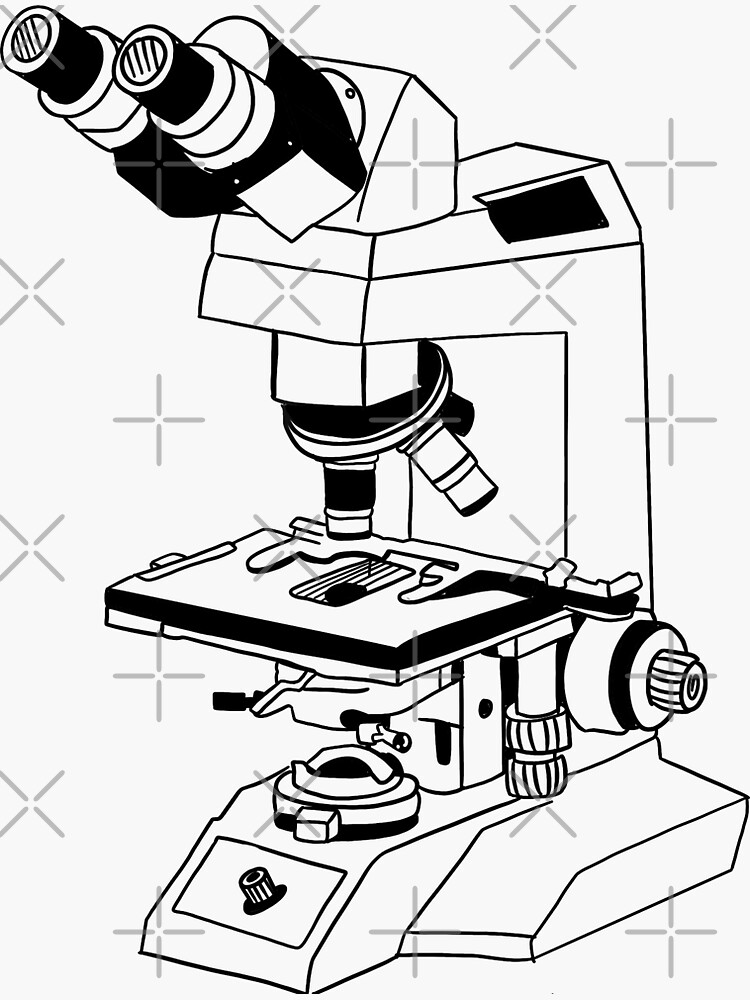This is a simple yet detailed black and white line drawing of a microscope, set against an off-white background. The illustration features two binocular-style eyepieces at the top, adorned with horizontal black lines. The main body of the microscope is depicted in a backward "C" shape, housing a rotating nosepiece with three different lenses of varying magnifications. Below the lenses, a slide holder is depicted, securing a rectangular slide that appears smudged, possibly with a sample like blood. The drawing also includes multiple adjustment knobs and screws for fine-tuning the focus, and a button at the base, possibly for a light source.

Overlaying the illustration, a series of gray X's and plus signs serve as a watermark, ensuring the image's protection. The meticulous attention to detail, despite its simplicity, captures the essential components and functionality of a traditional microscope, evocative of high school science classes.